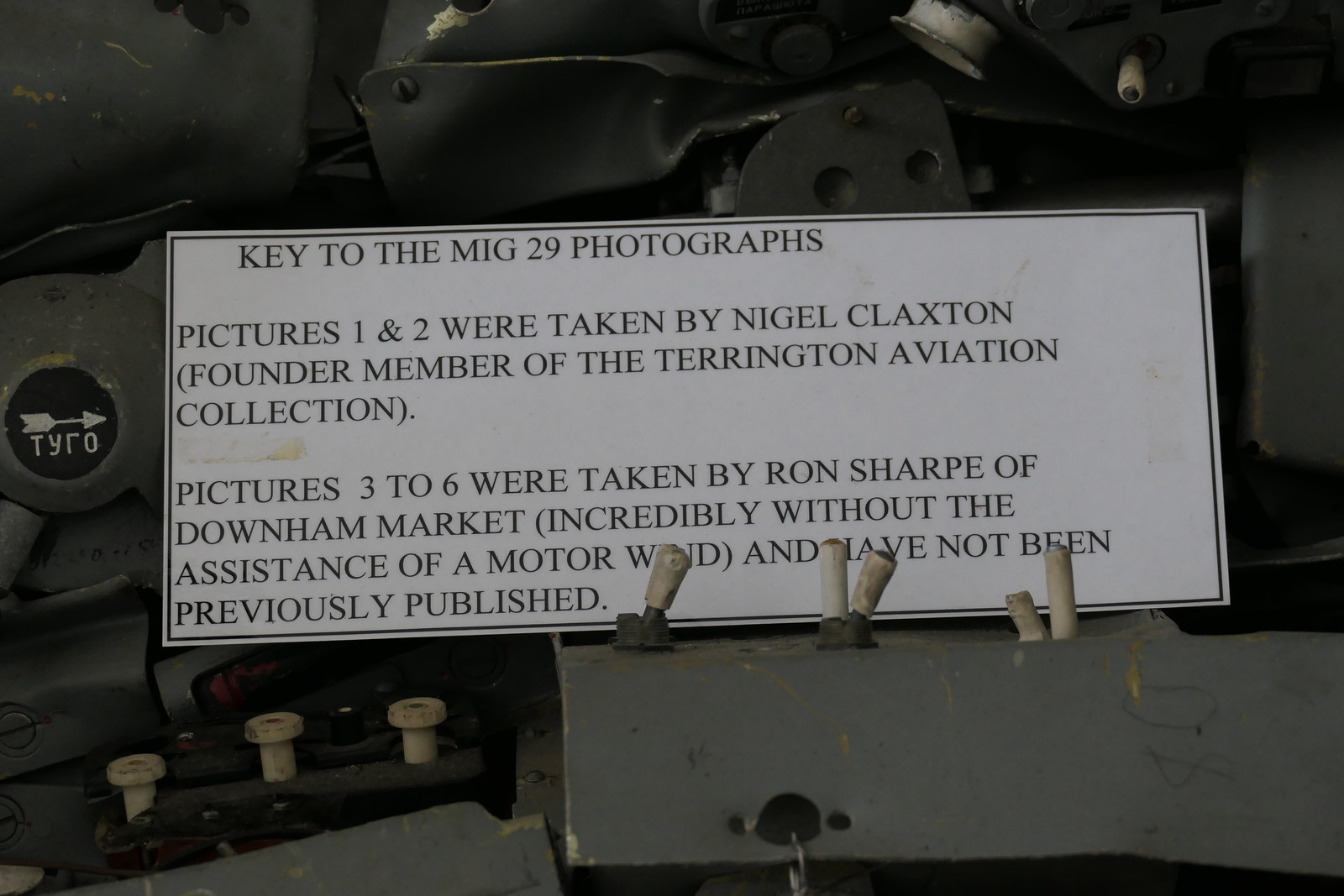The image is a color photograph in a landscape orientation showcasing a metallic gray rectangular machine adorned with an array of industrial components, including levers and buttons. Atop this mechanical contraption lies a white placard bordered in black. This placard, centered among the machinery, features black typography with the heading "Key to the MiG-29 Photographs." The text details that pictures one and two were taken by Nigel Claxton, a founding member of the Tarrington Aviation Collection, while pictures three to six were captured by Ron Sharp of Downham Market, remarkably without the assistance of a motor wind, and have not been previously published. Surrounding the placard are various mechanical parts and white controls, contributing to the industrial aesthetic of the scene.